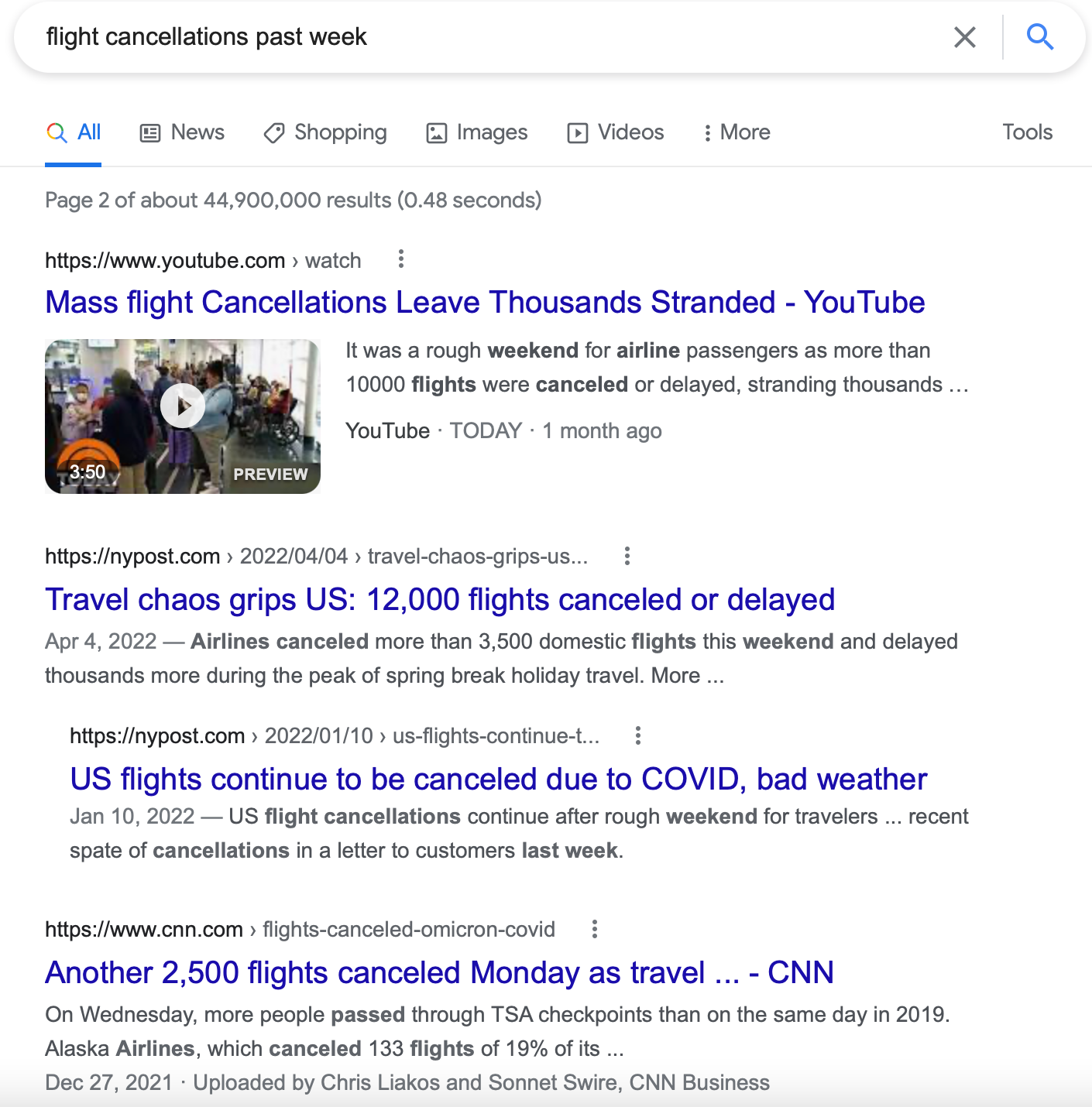Here's a cleaned-up, detailed caption for the image:

---

The image is a screenshot of a Google search results page. The user has searched for "flight cancellations in the past week." The browser is set to the "All" tab, highlighted among other tabs including News, Shopping, Images, Videos, and more. The page displays page 2 of approximately 44.9 million results. 

At the top of the search results is a YouTube video titled "Mass flight cancellations leave thousands stranded," accompanied by a preview thumbnail and a brief description. Followed by this, the next search result headline is from the New York Post: "Travel chaos grips US, 12,000 flights cancelled or delayed," with a descriptive snippet underneath. Another New York Post article is listed next, titled "US flights continue to be cancelled due to COVID, bad weather," also accompanied by a brief description. Further down, an article from CNN, "Another 2,500 flights cancelled Monday as travel...," is displayed with a summary from CNN.com.

The background of the image is white, maintaining a standard Google search aesthetic. Headline links appear in blue, while descriptions and URLs are in black text. Minor color highlights include red, green, and yellow icons within the "All" tab and search bar.

The predominant colors in the image are blue, black, and white, dotted with occasional red, green, and yellow elements. No additional browser profile details are visible.

---